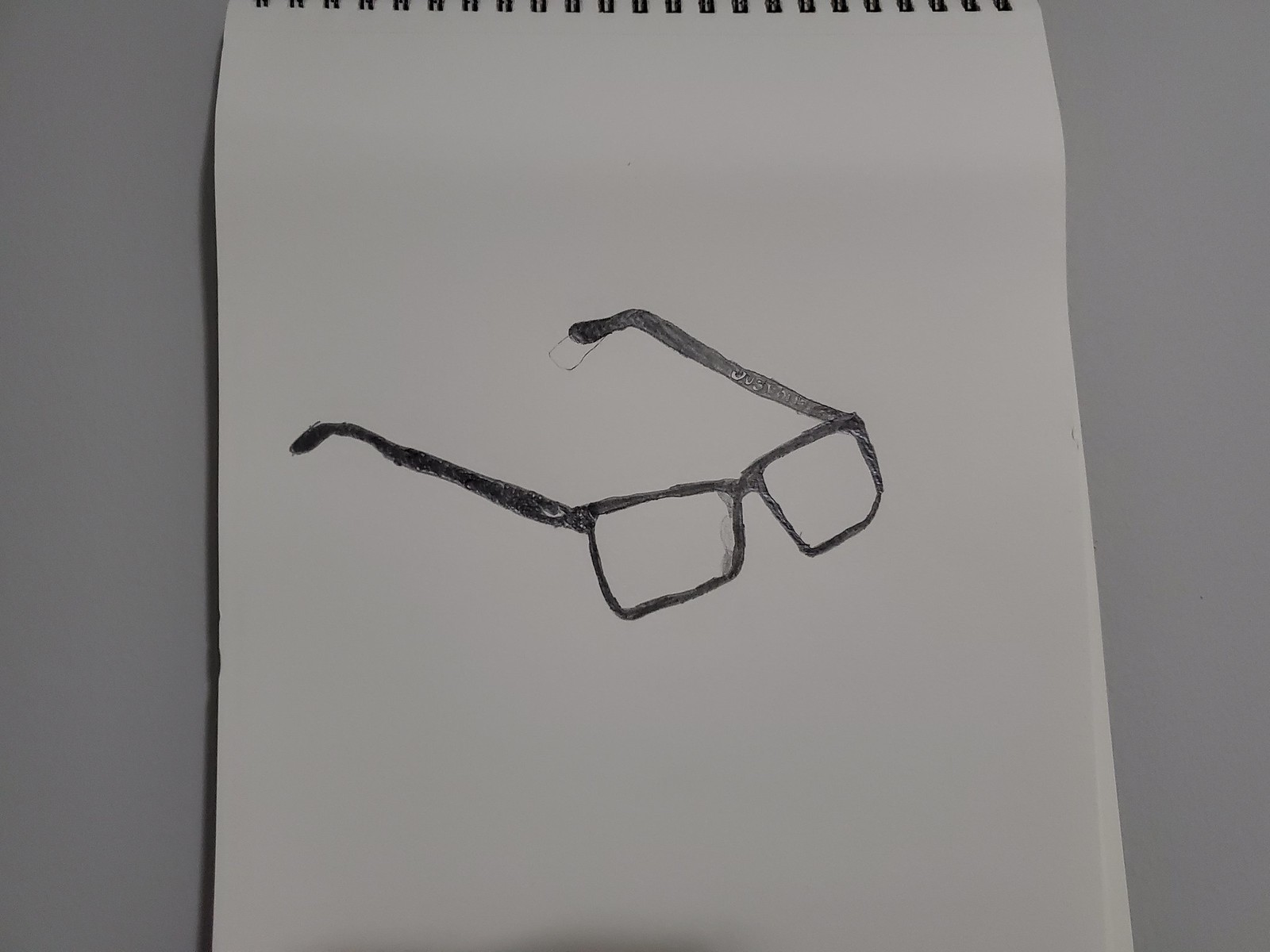This image captures a rough charcoal or pencil sketch on a slightly uneven piece of light gray paper, set against a solid dark gray background. The paper spans about three-fifths of the image from left to right, leaving dark gray borders on both sides. The sketch features a pair of black-framed spectacles drawn in a somewhat wonky, jagged style, suggesting the artist either lacked skill or rushed through the project. The glasses have rectangular lenses and visible nasal pads, but they appear beat-up and crooked, with smudges and signs of correction where previous lines were erased. Despite an attempt at three-dimensional shading, the overall drawing appears flat and imprecise, hinting at the artist's inexperience. The sketchpad's binding tines can be seen at the top, oriented vertically as if the pad were laid down on a hard surface.